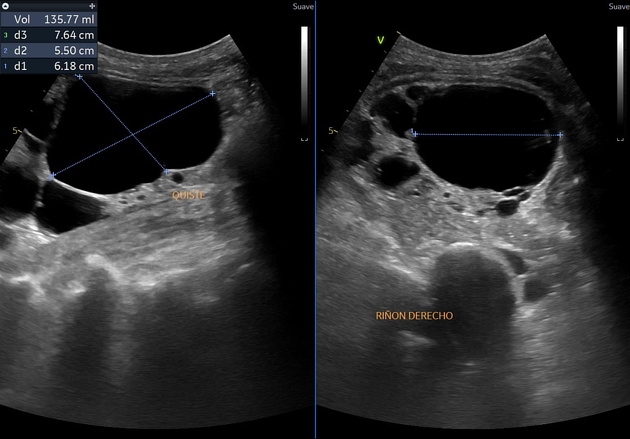This image presents what appears to be two side-by-side medical scans—potentially ultrasound or radiology images—of an individual's abdominal area. The left scan features intersecting lines creating an X within a black area, with measurement data on the periphery: Volume 135.77 milliliters, D3 at 7.64 centimeters, D2 at 5.50 centimeters, and D1 at 6.18 centimeters. The label "Quiste" is visible, suggesting the presence of a cyst. A similar blue line is drawn across the upper part of this scan, with the label "Rinonderecho" or "Derecho."

The right scan displays what might be the shape of a human head or potentially a tumor, yet the rest of the body is obscured. There are additional markings including a blue line between two plus signs and a green 'V'. Key numbers include five and the duplicate label "Rinonderecho." The collective details and shared elements point to a thorough investigation of potential abnormalities in the abdominal region, with a strong possibility of a cyst and ambiguous other formations.